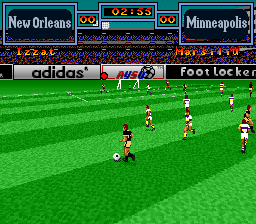This square-shaped image is a screenshot from an old-style 64-bit soccer game. Set on a vibrant green, pixelated grass field with distinct white lines, the visual captures the essence of retro gaming. The field features players from two teams: one team in black jerseys paired with yellow shorts and black socks, and another in white shirts marked with a maroon stripe and matching white shorts.

In the background of the field, the top left corner shows a blue rectangular box labeled "New Orleans" in white text, while the top right corner similarly displays "Minneapolis" in blue. Centrally positioned at the top is a scoreboard with bold red and yellow elements, reading "2:55" into the game with both teams tied at a score of 0-0.

Around the edges of the field, several banners and advertisements add to the nostalgic atmosphere. Prominent ads include "Adidas" in bold black letters, "AYSO" in red and blue, and "Foot Locker." One banner features a football graphic, though its affiliated logo remains unclear. The audience is faintly visible beyond the field, providing a backdrop of spectators intently watching the action unfold.